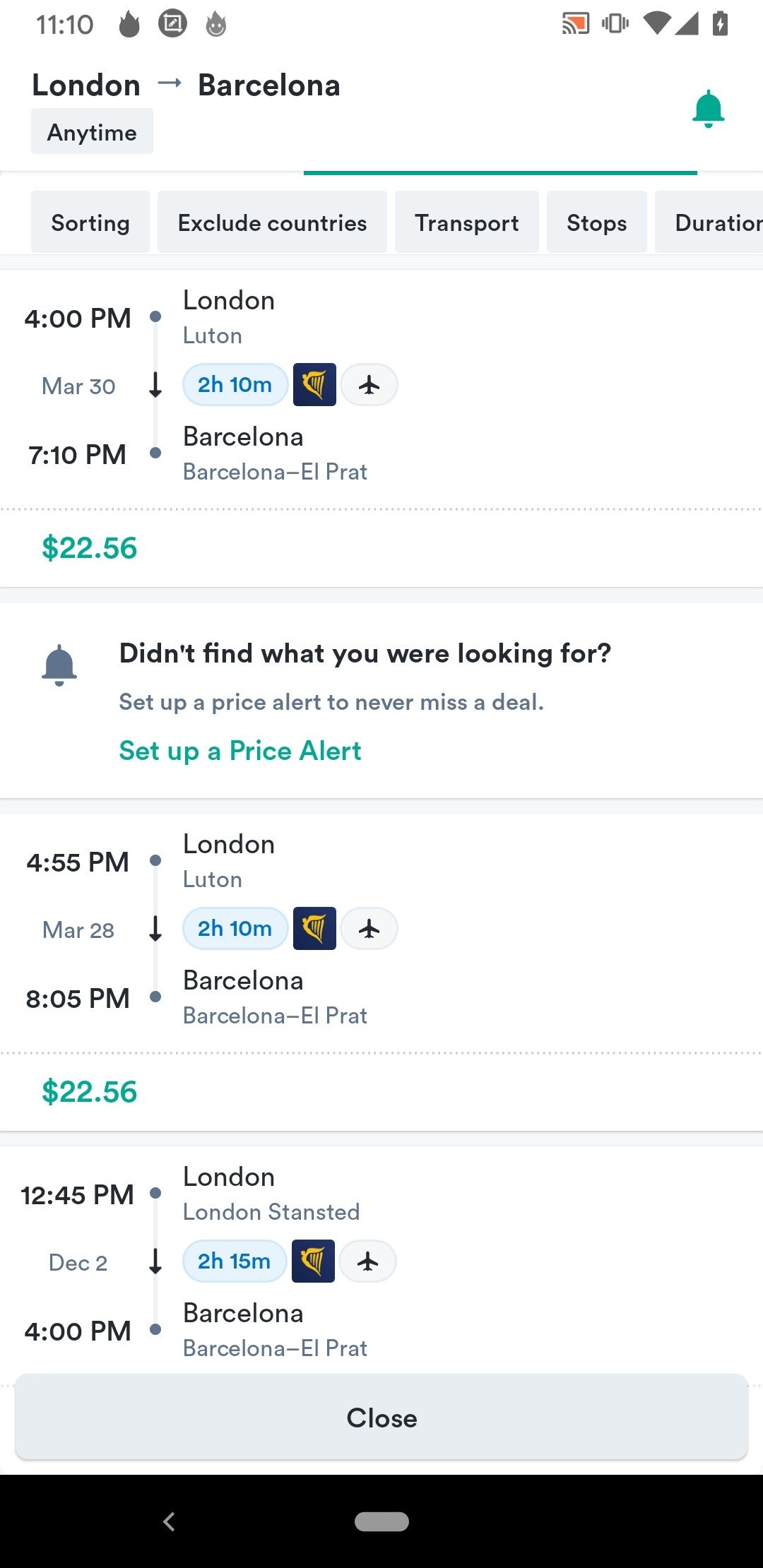Here is a detailed and cleaned-up descriptive caption for the image:

---

The screenshot depicts a smartphone interface captured at 11:10 AM. At the top left corner, there are two fire icons, one of which includes a smiley face. Adjacent to these is a pencil-in-a-box icon. Despite showing full Wi-Fi bars, there is an error message indicating a malfunction with the Wi-Fi connectivity. The phone is in vibrate mode, shows full signal bars, and the battery is fully charged.

Displayed prominently on the screen is a travel itinerary with options for a journey from London to Barcelona. It offers multiple modes of transport and shows specific details such as sorting options, which include excluding countries, transport stops, and journey duration.

One travel option listed shows a trip from London to Luton on March 30th, departing at 4 PM and arriving at Barcelona Alparet at 7:10 PM, totaling a duration of 2 hours and 10 minutes, with a fare of $22.56. 

Another option details a journey from London to Luton, departing at 4:55 PM and arriving at 8:05 PM, again to Barcelona Alparet, with the same fare of $22.56. 

A further option highlights a trip from London Stansted, departing on December 2nd and arriving in Barcelona after a 2-hour and 15-minute duration.

A notification bell with a green indicator suggests there is an unread alert. There is also a green text prompt to "Set up a price alert and never miss a deal," encouraging the user to stay updated on prices.

At the bottom of the screen, typical smartphone navigation buttons are visible: home, menu, and back. However, the conventional menu button is missing.

---